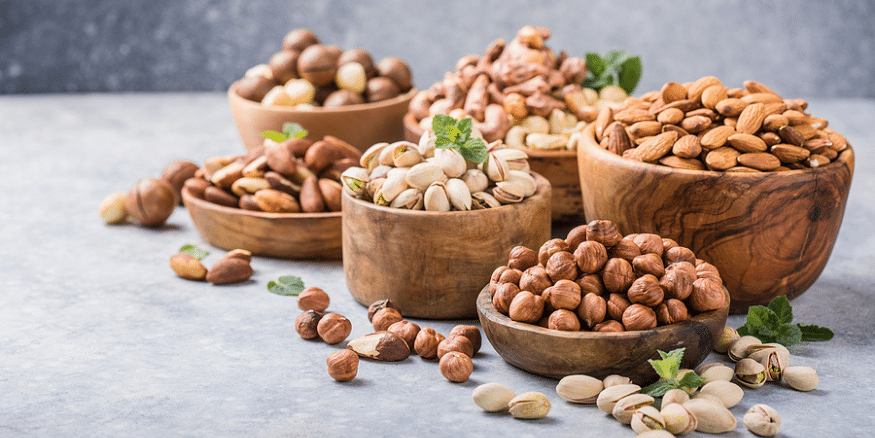This image depicts a collection of six intricately carved, light brown wooden bowls, each overflowing with a variety of nuts, arranged on a lightly blue-toned, grayish table. The bowls vary in size from shallow dishes to small, cup-like containers. The front-most bowl is a short, inch-tall wooden bowl brimming with walnuts, while to its rear stands a bowl about three times taller, filled to the top with pecans. The other bowls contain an assortment of nuts, including almonds, pistachios, macadamia nuts, hazelnuts, and cashews, easily identifiable by their distinct shapes and textures. The nuts extend beyond the bowls, with around 15 to 20 scattered artistically on the table surface. Some bowls also contain sprigs of green spearmint or peppermint, adding a touch of freshness to the display. In the background, a blur hints at a sparkly, dark wall, enhancing the focus on the earthy tones of the nuts and bowls. The empty left side of the table contrasts with the rich, bustling arrangement of wooden bowls on the right, creating a balanced yet dynamic visual composition.